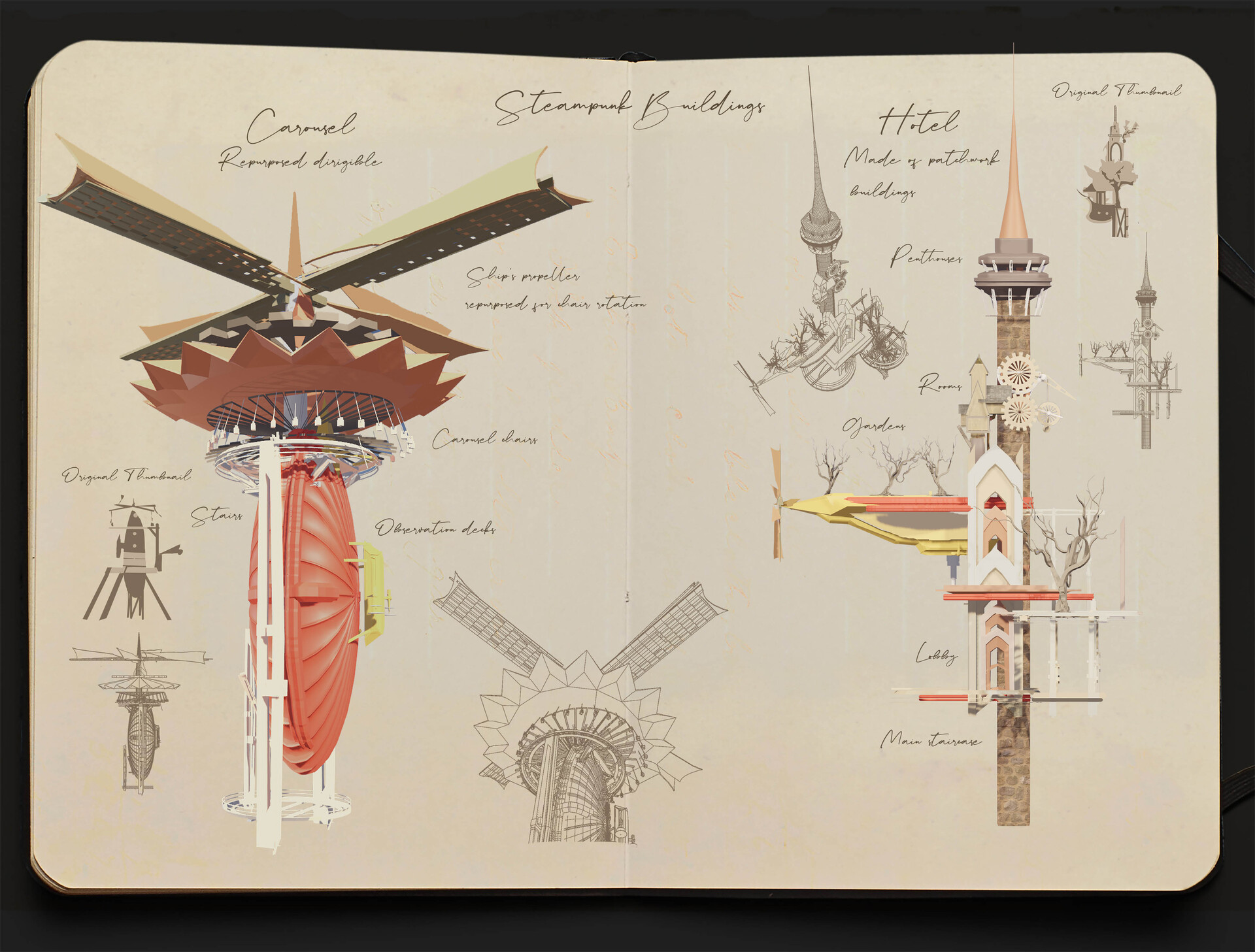This is a color photograph of an open sketchbook featuring intricate steampunk-themed designs. At the top, the title "Steampunk Buildings" is inscribed in cursive. Towards the left side of the page, there is a detailed color drawing of a carousel labeled "Revamped Dirigible," surrounded by complex steampunk machinery. Adjacent to this main drawing are smaller black-and-white or sepia-toned thumbnail sketches depicting the preliminary concepts.

On the right side of the sketchbook is an elaborate illustration of a slender, pointy tower reminiscent of a space needle intermixed with elements of a church. This structure is depicted in beige, gray, and pink tones, with peach and yellow shelves extending from it, bearing what appear to be trees—an intriguing blend of nature and machinery typical of steampunk aesthetics. Gears and other ornamental details enhance the fantastical appearance. Scattered around this main drawing are more miniature sketches that showcase various angles and intricate parts of the design, providing further insight into the artist's vision. The entire sketchbook page is richly detailed, presenting a fascinating collection of steampunk architectural concepts that could easily find their way into a comic book or graphic novel.